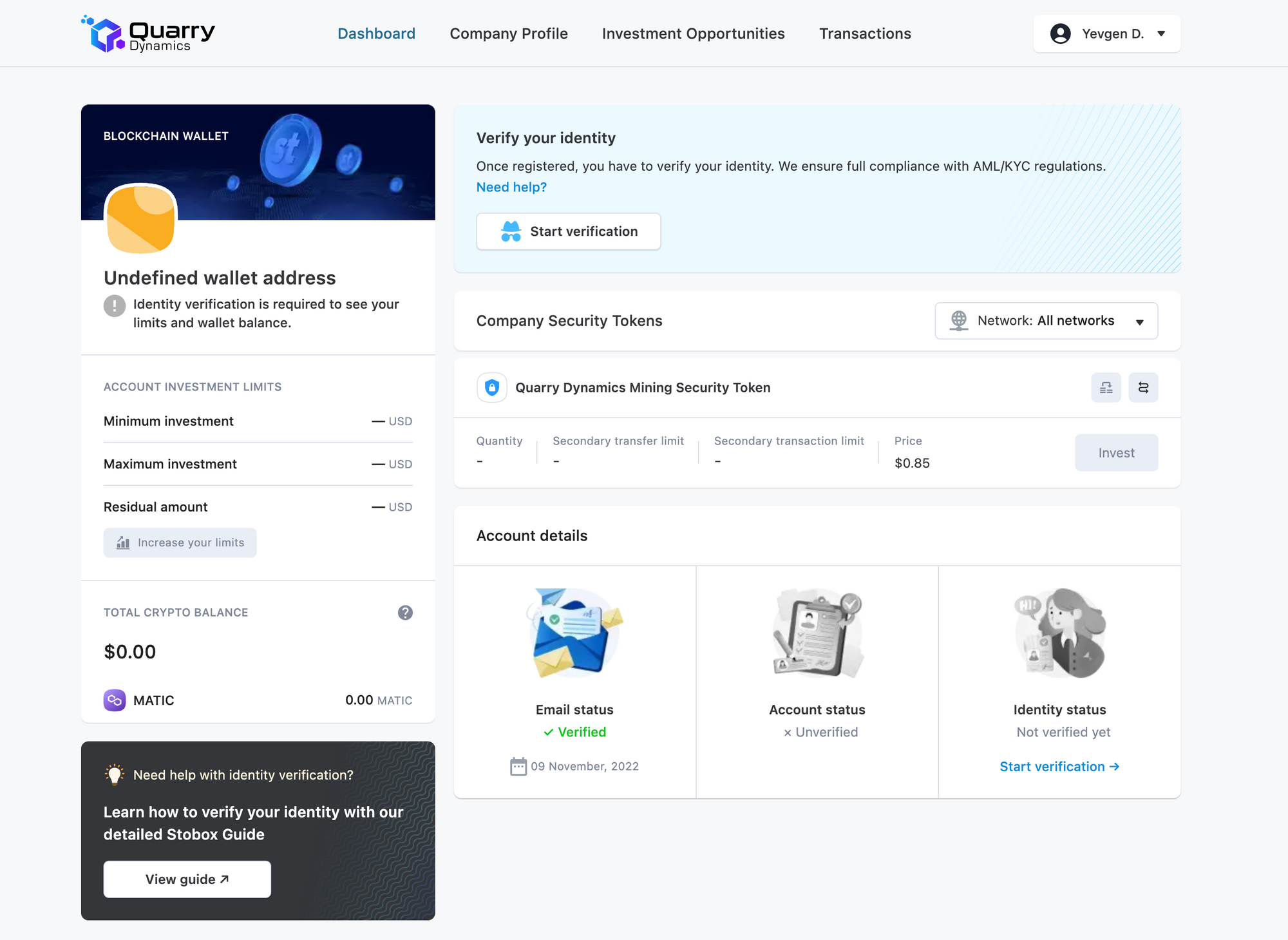The webpage in the image appears to be from Quarry Dynamics. In the top left corner, the Quarry Dynamics logo is prominently displayed. Below the logo, there is a navigation bar with "Dashboard" highlighted in blue, while "Company Profile," "Investment Opportunities," and "Transactions" are listed in black.

In the top right corner, there is a drop-down menu that reads "Yevgen D." 

The right-hand side of the screen is dominated by a box titled "Blockchain Wallet." This section mentions that an "undefined wallet address" requires identity verification to view limits and wallet balance. It also details account investment limits, including minimum investment, maximum investment, and residual amount, but these fields are not populated. The "Total Crypto Balance" is shown as zero.

In the bottom left corner, there is a black box featuring a light bulb icon. This section offers help with identity verification, linking to the Stobox guide through a white, rectangular button labeled "View Guide."

The central part of the image, taking up the majority of the page, includes a section titled "Verify Your Identity." It explains the need to verify identity upon registration to comply with AML/KYC regulations. There is a prompt asking "Need help?" with a button to "Start Verification."

Further down, another section is dedicated to "Company Security Tokens," specifically the Quarry Dynamics Mining Security Token. It lists the details such as Quantity, Secondary Transfer Limit, and Secondary Transaction Limit, all of which are undefined, and notes the price as $0.85.

At the bottom of the page, it shows "Account Details," with "Email Status" marked as verified (highlighted in green with a check mark). However, "Account Status" and "Identity Status" are marked as unverified, with a prompt to "Start Verification."